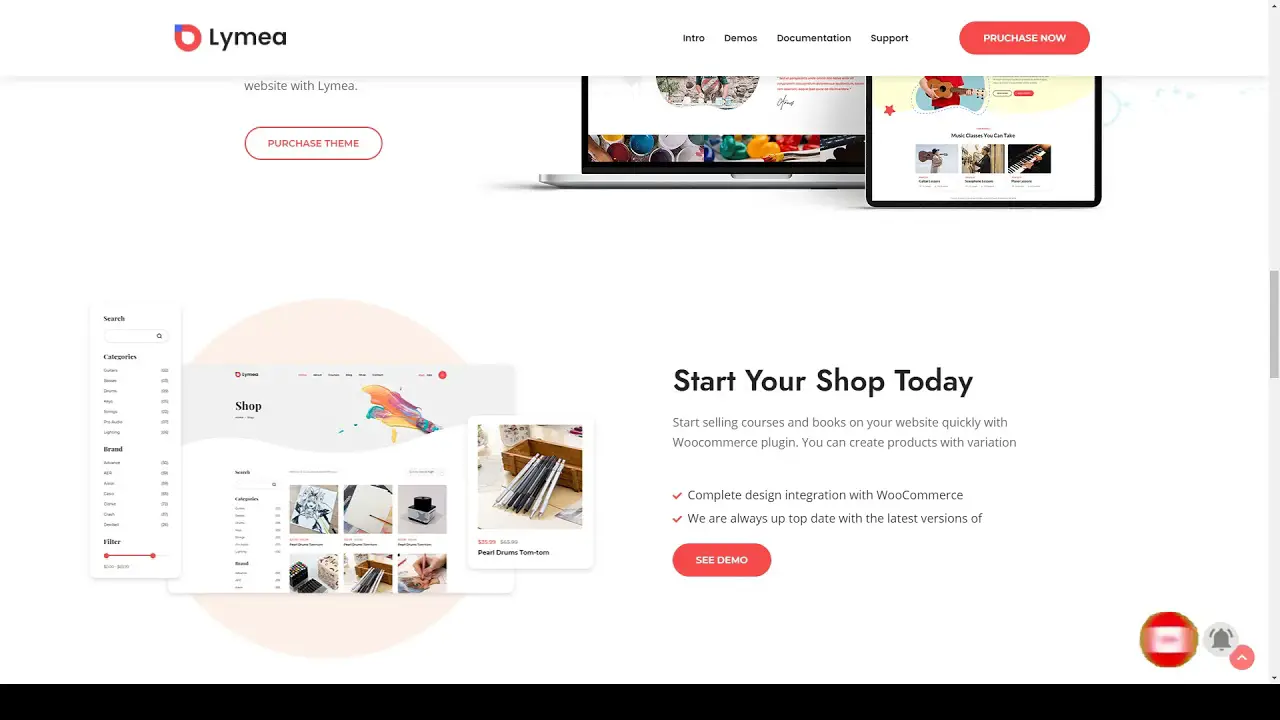This is a screenshot of a web application or website named "Limea" (spelled L-Y-E-M-E-A). To the right of the screen, there are four selectable informational tabs labeled: Intro, Demos, Documentaries, and Support. Below these tabs, a prominent red "Purchase Now" button is clearly visible. In the main viewing pane, there is information detailing the process of starting your shop today, suggesting that this platform is tailored for creating online shopping or selling websites. On the left side of the screen, there is an image showcasing an example web page layout. Additionally, there is a button that allows users to view another demo. Overall, this appears to be a web interface design software specifically designed for building e-commerce or shopping websites.